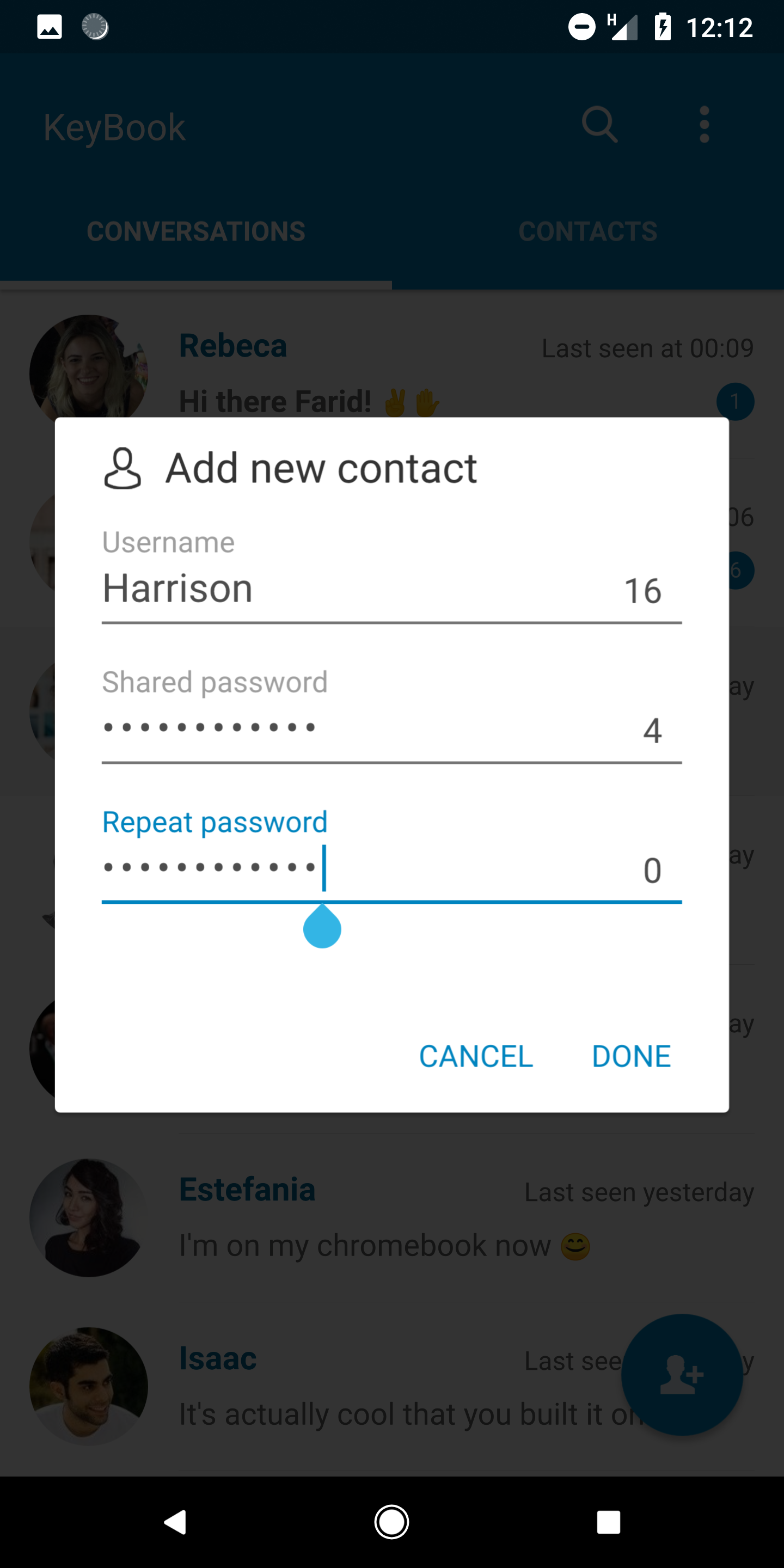The image displays a smartphone screenshot with the time indicated at 12:12 PM. The signal strength is shown as two out of four bars, and the battery indicator is almost full. The background image appears to be gray and indistinct. The app open on the screen is named "Keybook," as indicated in the top-left corner. The primary interface shows a list of conversations and contacts, each with a profile picture, the contact's name to the right, and a snippet of the last text message beneath the name. Notably, the top contact has a different date for 'last seen' compared to others, which read "last seen yesterday."

Centrally located is a white square overlay with options for adding a new contact. At the top of this overlay, there is a header that reads "Add New Contact." Beneath this, the text fields prompt for a "Username" with a placeholder, "Harrison 16," and then for a "Shared Password," which is obscured by asterisks. Below these fields are two buttons labeled "Cancel" and "Done."